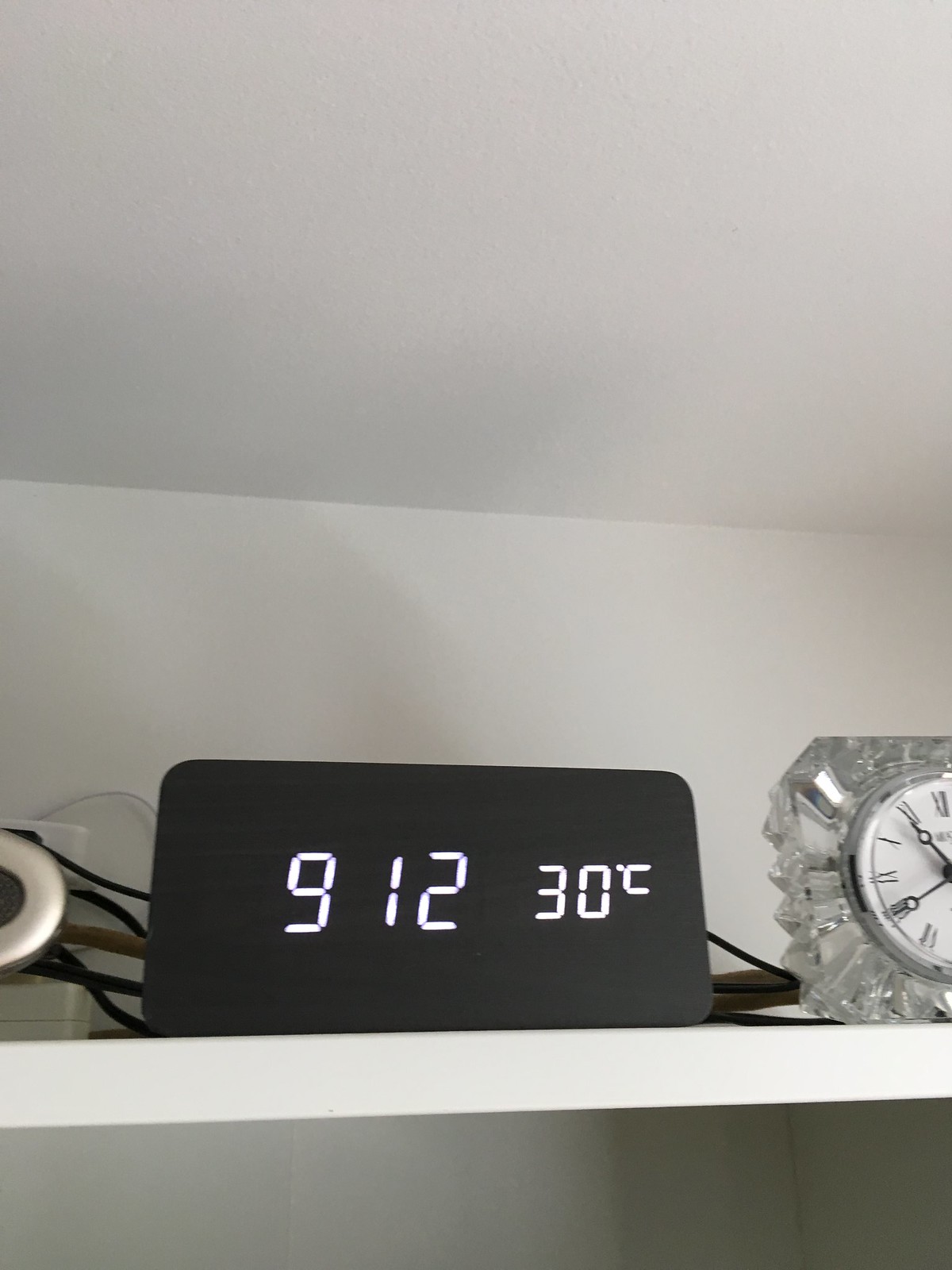This image showcases a crisp, white shelf set against an entirely white backdrop, encompassing both the wall and the slanted ceiling above. Centrally positioned on the shelf sits a sleek, black alarm clock displaying the time as 9:12 and the temperature as 30 degrees Celsius in white digital numbers. To the right of the alarm clock, partially eclipsed, is a sophisticated clock with a clear, crystalline exterior. The clock face is white with black hands ending in circular tips and features Roman numerals. Behind this clock, a black cord is visible, intertwined with an indistinguishable brown object. On the left side of the alarm clock, additional black cords are noticeable alongside more of the brown item, accompanied by a silver circular object adorned with dots at its center. Beneath this arrangement lies a tan-colored element, completing the meticulously arranged scene on the pristine shelf.